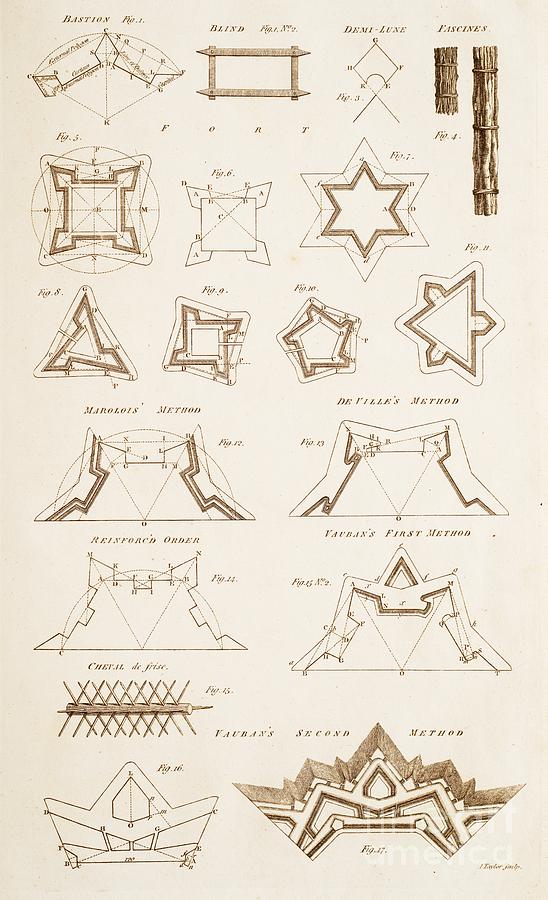This illustration possesses an antique quality, resembling a detailed engraving from an old manuscript. The parchment is a light brown, tan hue, adding to its vintage charm. In the intricate image, there is a collection of various geometric diagrams, each meticulously drawn and labeled with figure numbers. The accompanying text is challenging to decipher due to its small size and elaborate font. Nestled among the geometric shapes, two prominent illustrations depict wooden structures. These constructions, possibly archaic weapons or defensive fortifications, hint at medieval military engineering and evoke the protective strategies of castles or fortresses. The overall scene conveys a blend of mathematical precision and historical context, transporting the viewer to a bygone era of scholarly exploration and strategic innovation.